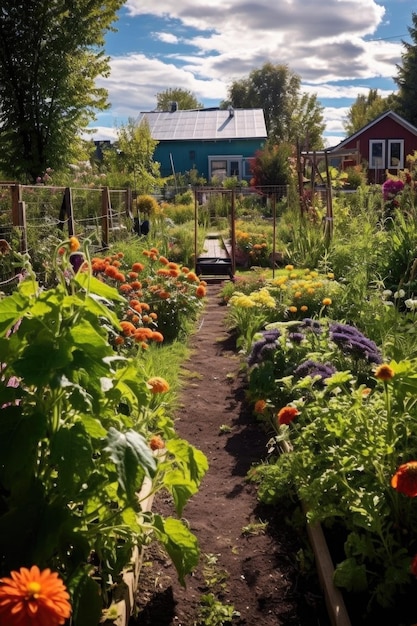This vibrant outdoor photograph, displayed in a portrait orientation, captures a meticulously maintained garden nursery viewed from a dirt path lined with flowering plants. In the foreground, rows of flowering green plants, predominantly orange zinnia flowers with yellow centers, are neatly arranged in slightly elevated wooden crates and planters on either side of the path. On the left, the garden is bordered by a sturdy wooden fence with tall posts and mesh metal. Walking down the path, one encounters a blue building, possibly a house or potting shed, boasting blue siding, a light gray roof with a low chimney on the right, and it's complimented by an adjacent dark red structure. Tall trees with lush green foliage tower in the background under a bright blue sky adorned with heavy white clouds. A standout feature includes a prominent bloom of orange flowers in the lower corners, augmenting the vivid, colorful representation of this well-tended garden space characterized by photographic realism.